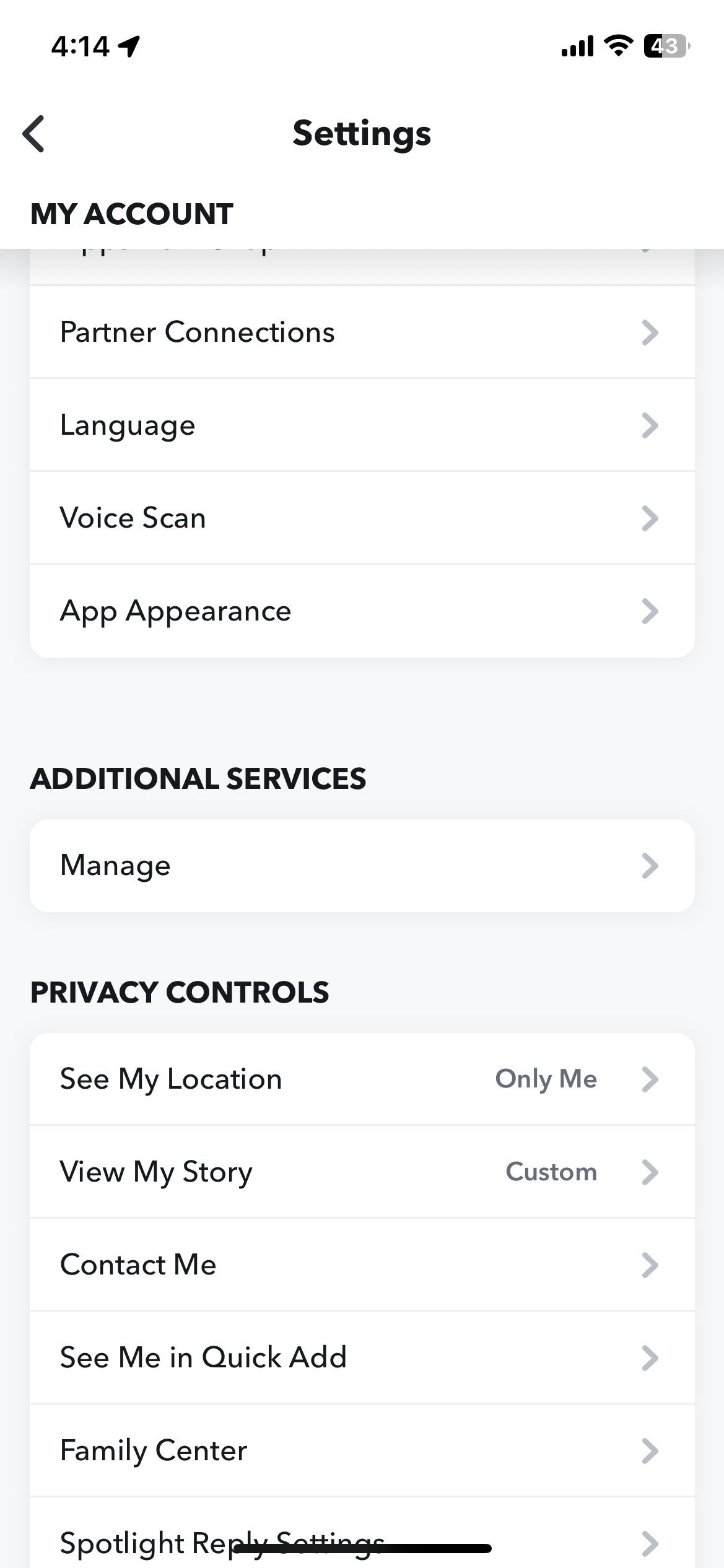A detailed screenshot of a smartphone's settings page is displayed. In the upper left corner, the time is shown as "4:14" alongside a small arrow pointing left. On the upper right corner, status indicators show full cellular signal bars, an internet connection icon, and the battery percentage at 43%.

Centrally positioned at the top of the screen, "Settings" is written in bold black text, accompanied by a left-facing arrow icon to its left. Just below, left-aligned and capitalized in black, the label "MY ACCOUNT" appears. Under this, a series of options are listed, each with an arrow pointing to the right:
1. "Partner Connections"
2. "Language"
3. "Voice Scan"
4. "App Appearance"

A space separates these options from a new section titled "ADDITIONAL SERVICES," also in bold and all caps. Below this, a single option labeled "Manage" is accompanied by an arrow to the right.

The next section is "PRIVACY CONTROLS," also in bold and all caps. The options under this section include:
1. "See My Location" - labeled "Only Me" next to the arrow on the right.
2. "View My Story" - labeled "Custom" next to the arrow.
3. "Contact Me"
4. "See Me in Quick Add"
5. "Family Center"
6. "Spotlight Replay Settings"

A black bar crosses horizontally through the word "Replay," running from the 'P' in "Spotlight" across to the end of "Replay."

The overall design is minimalist with a light gray background and black text, making the interface clean and uncluttered. Key headers such as "Settings," "MY ACCOUNT," "ADDITIONAL SERVICES," and "PRIVACY CONTROLS" use bolder and darker typography, while descriptive text remains in a standard font. Each word is capitalized except for the word "in," which stands out in lowercase.